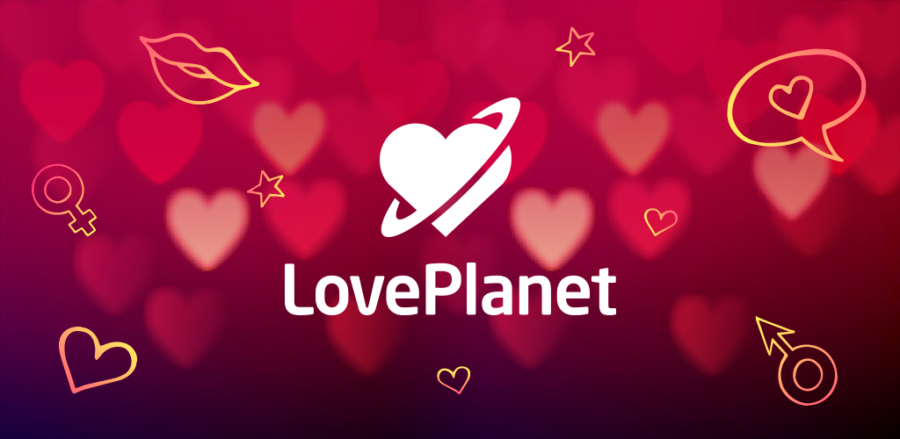The image showcases a vibrant graphic art piece for a company or product named "Love Planet," prominently featuring the name "Love Planet" in capitalized white lettering at the center. Above the text, there is a distinctive logo comprising a white heart encircled by a ring reminiscent of Saturn. The background of the image is a striking color gradient that transitions from deep black at the bottom to a rich red at the top, giving a dynamic visual effect. Scattered throughout this background are multiple overlapping and blurry hearts in varying shades of pink to red, enhancing the theme of love and affection.

Adding to the intricate design, numerous yellow icons are dispersed around the main elements. These include gender symbols, stars, small hearts, a pair of lips, and a speech bubble containing a heart, all contributing to the whimsical and inclusive atmosphere. The overall composition effectively blends these diverse elements, creating a cohesive and eye-catching graphic that celebrates love in its many forms.